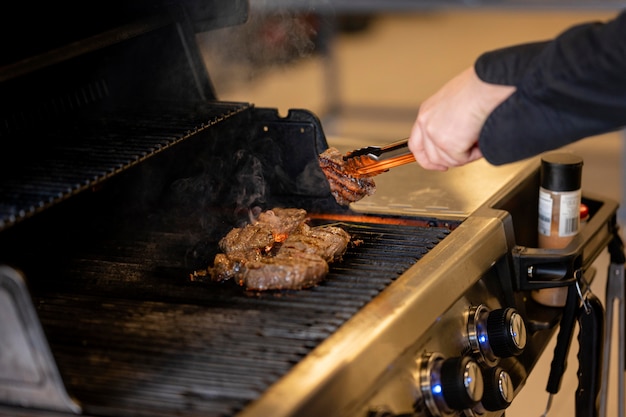In this photo, a person is grilling a couple of hamburgers. The grill is open, displaying several pieces of meat being smoked, with smoke visibly rising from the grill. The individual, wearing a long-sleeved black shirt, is holding a pair of tongs, either flipping or moving one of the burgers. Their hand and the lower part of their arm are clearly visible.

The grill itself is a combination of black and gold colors, featuring black knobs with silver centers on the front. The side handle of the grill holds an assortment of utensils and spices, including a spray can likely containing oil to prevent food from sticking. The cooking setup appears detailed and organized with condiments ready to be applied to the food. Charcoal can be seen in the background, adding to the authentic grilling atmosphere. It's a vivid scene of someone diligently grilling on a hot summer day, putting the finishing touches on a batch of delicious-looking burgers.